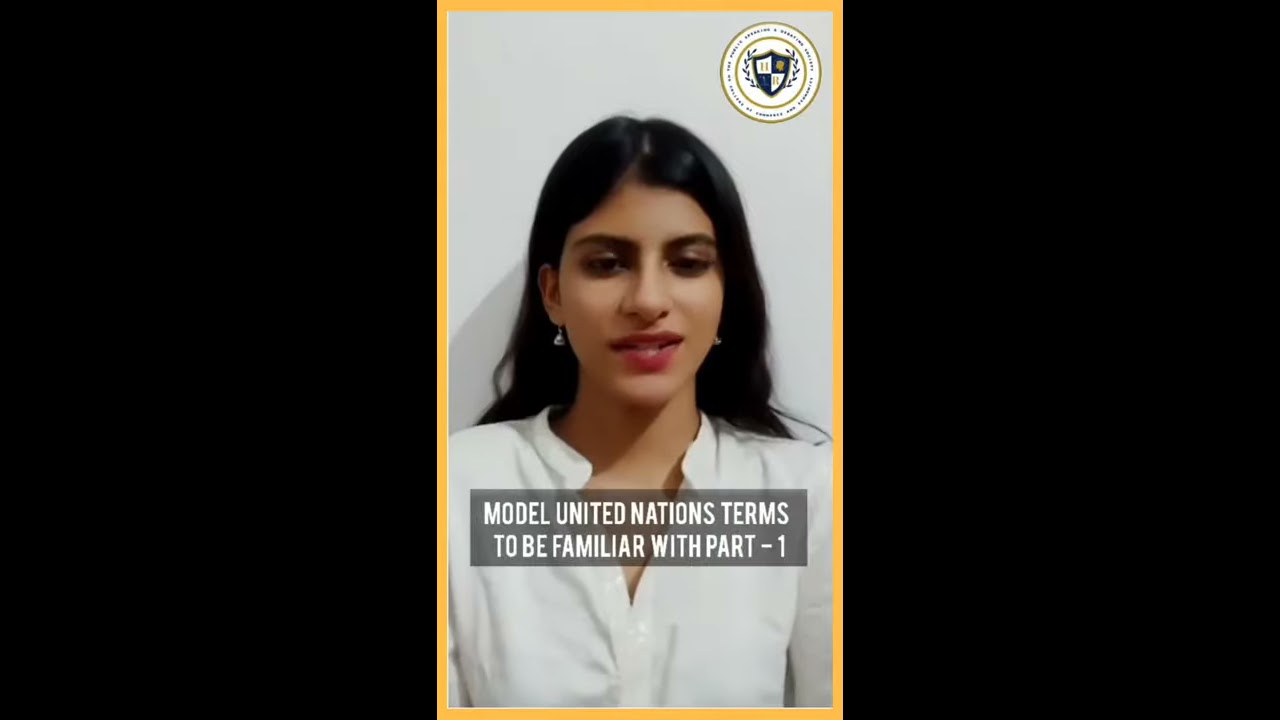The image displays a woman with black, middle-parted hair and dark eyes, smiling slightly, with small earrings and red lips. She is wearing a white button-down shirt with no collar, standing against a stark white background. The central portion of the image, outlined in orange with black borders on both sides, features a gray banner superimposed across her chest, reading "Model United Nations Terms to Be Familiar With Part-1" in white, capitalized text. In the upper right corner, there is a circular logo with blue, white, and gold elements, possibly a shield, adding a formal touch to the presentation.